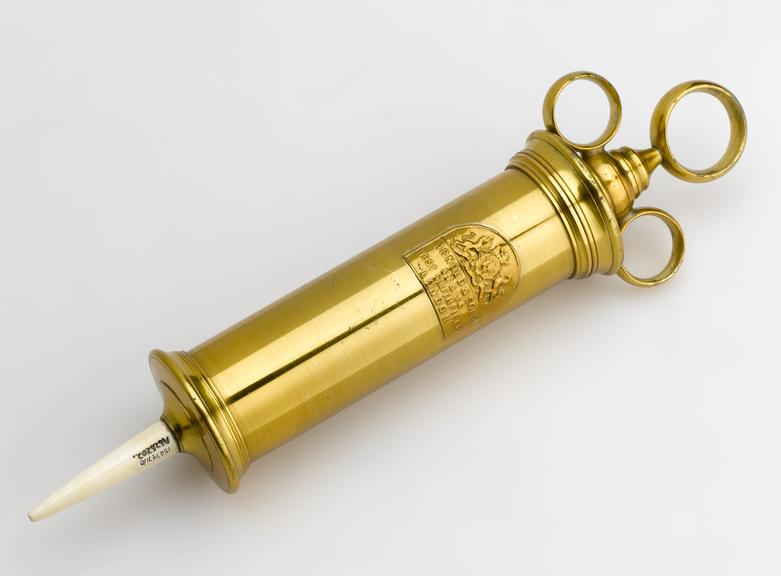The image features a color photograph of an antique brass syringe, displayed against a creamy white background. The syringe, which is the focal point of the picture, stretches diagonally from the bottom left to the top right. At the bottom left, the syringe has a flexible, white plastic tip or cap, likely not original to its design and featuring some large, unreadable writing. The main body of the syringe is a thick, cylindrical, golden brass tube, polished to a bright sheen and adorned in the middle with a detailed, yet indistinguishable, engraved heraldry symbol and some text. This intricate ornamentation gives the piece a distinctly vintage appearance. On the top end of the syringe, there are three round metal rings: two on each side and one larger central ring. These rings are part of the mechanism, designed for the user to insert fingers through the side rings and press down on the central ring to eject the contents, making it potentially useful for administering medicine to animals. The overall aesthetic is both functional and ornamental, suggesting it is an elegantly crafted yet practical tool from a bygone era.